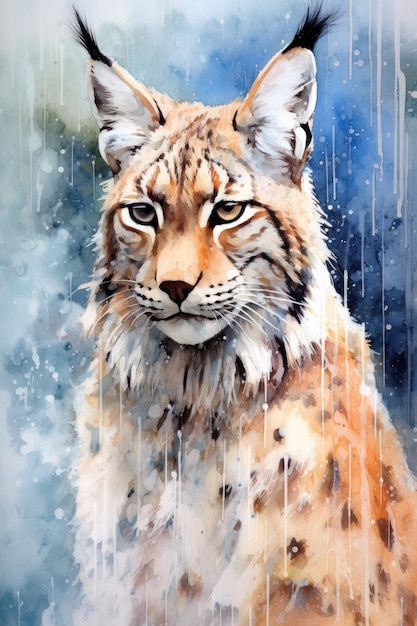In this watercolor painting, a fox with vivid red fur and golden eyes stands in the rain, its wet fur showing touches of white. Subtle black stripes and spots accentuate the fox's head and around its eyes, adding to the detailed definition of its face and ears. The animal's fur appears more blurry and undefined on its body, creating a sense of motion. The background features a cloudy mixture of blue, green, and gray with hints of pink, evoking a foggy, smoky atmosphere. Raindrops, depicted with brushstrokes, fall around the fox, which looks out into the distance, possibly searching for prey as it stands vigilant, seemingly moving slightly in the rain.